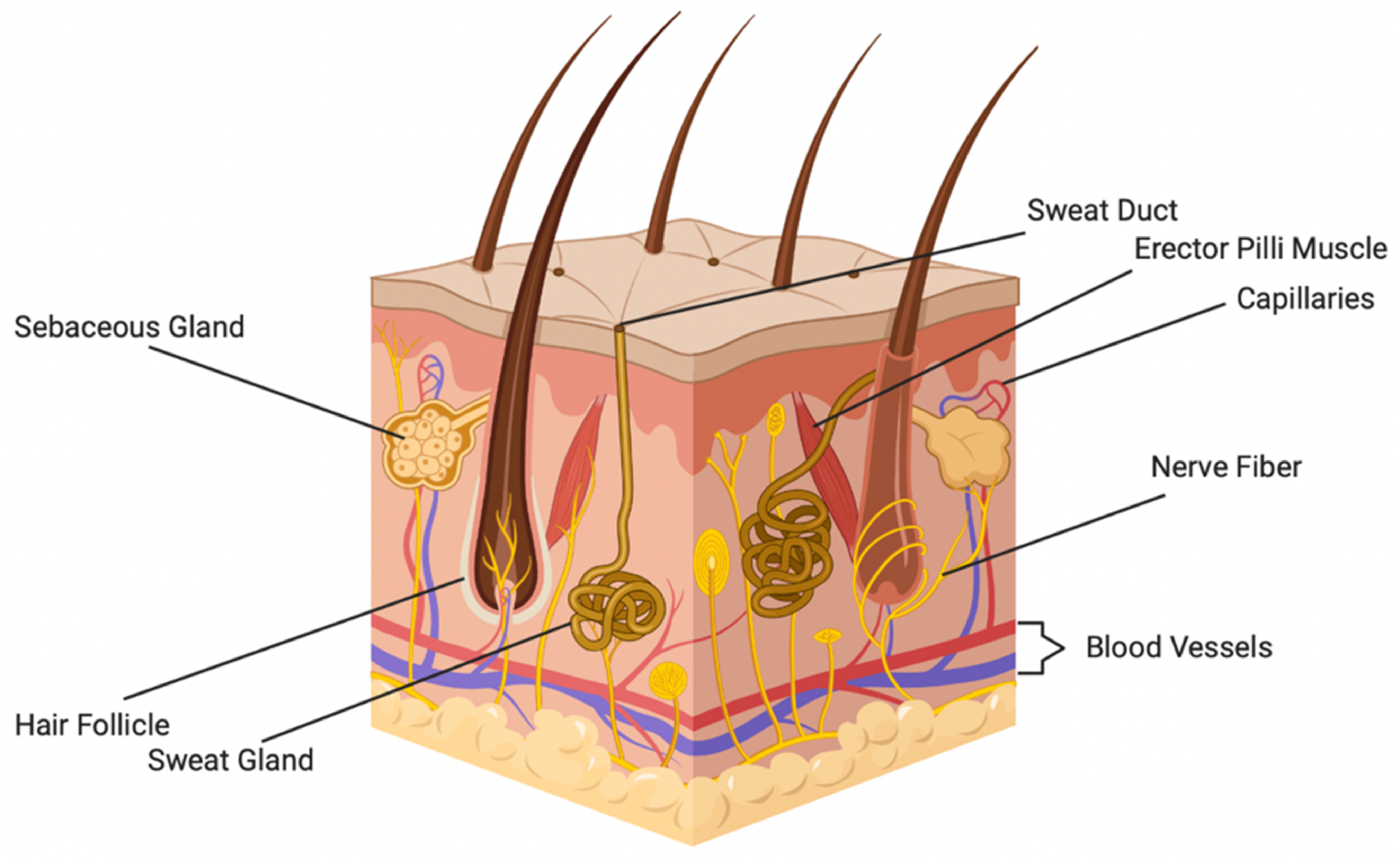The image depicts a detailed and colorful digital drawing of human skin in landscape mode, showcasing its various anatomical structures. The top of the image features a tan flat layer with brown hair follicles protruding from it. Below this surface, multiple structures are intricately labeled. On the left side, lines point to the sebaceous gland, hair follicle, and sweat gland, each highlighted in different shades of brown. The bottom center portion is filled with numerous small yellow circles, representing adipose tissue or fat cells. The right-hand side labels include blood vessels marked by red and blue lines, nerve fibers indicated by thin yellow lines, and capillaries shown by red thin lines. Further up, a line points to the erector pili muscle, depicted as a red leaf-like structure in the center, and at the very top, a sweat duct is labeled. The diagram comprehensively illustrates the layered and structural complexity of human skin, from the roots of the hair to the various glands and vessels embedded within.